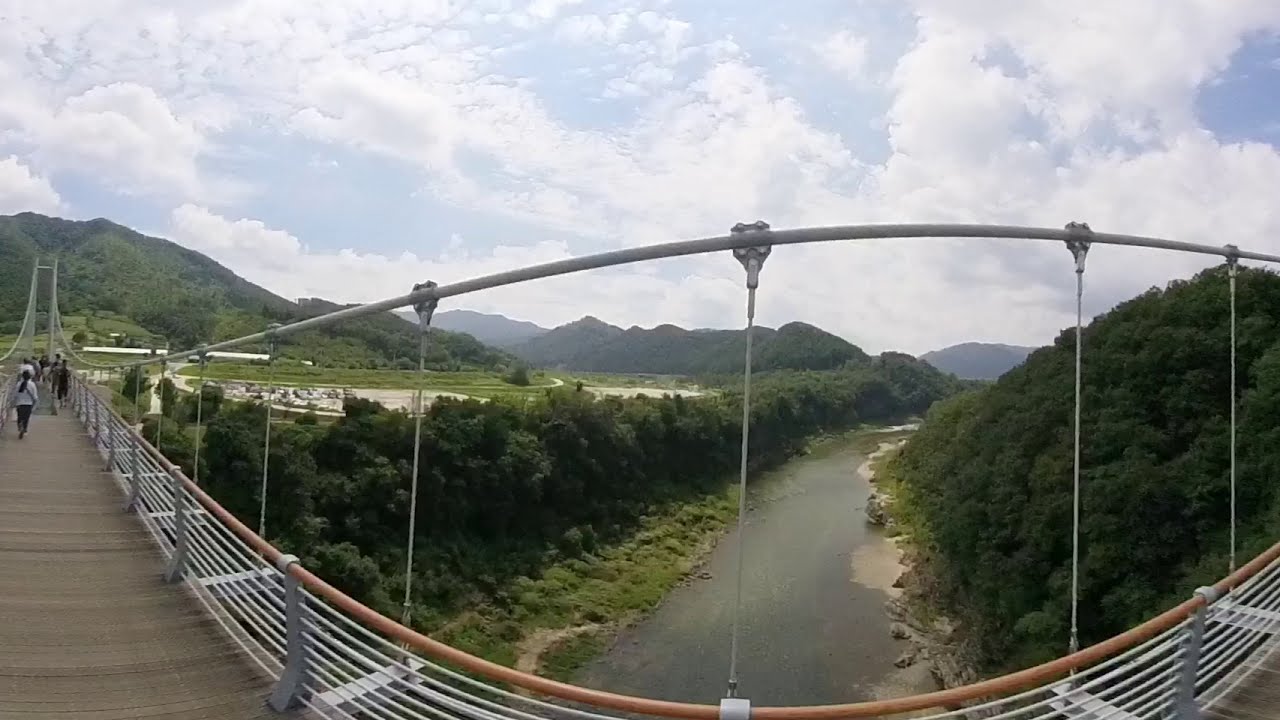This outdoor image, captured with a wide fish-eye lens, features a suspension bridge high above a slow-flowing stream or river. The water below appears dark gray, with minimal rapids. The bridge's railings are primarily metallic silver, with a copper-colored handrail and smaller tubular aluminum railings beneath. In the foreground, the bridge curves upward slightly before descending, and you can see numerous people walking along it toward the left. 

To the right of the stream, there's a small sandy beach area, quickly giving way to dense greenery consisting of trees and bushes. On the left, a similar row of trees lines the riverbank. Beyond the bridge and stream, a lush hill covered in green grass and trees rises, with more tree-covered hills and potential mountain ranges visible in the far distance.

In the background, the sky is a pale blue filled with scattered clouds. Some distant buildings can be seen on the left. Overall, the scene exudes a tranquil, natural beauty amidst the constructed bridge.